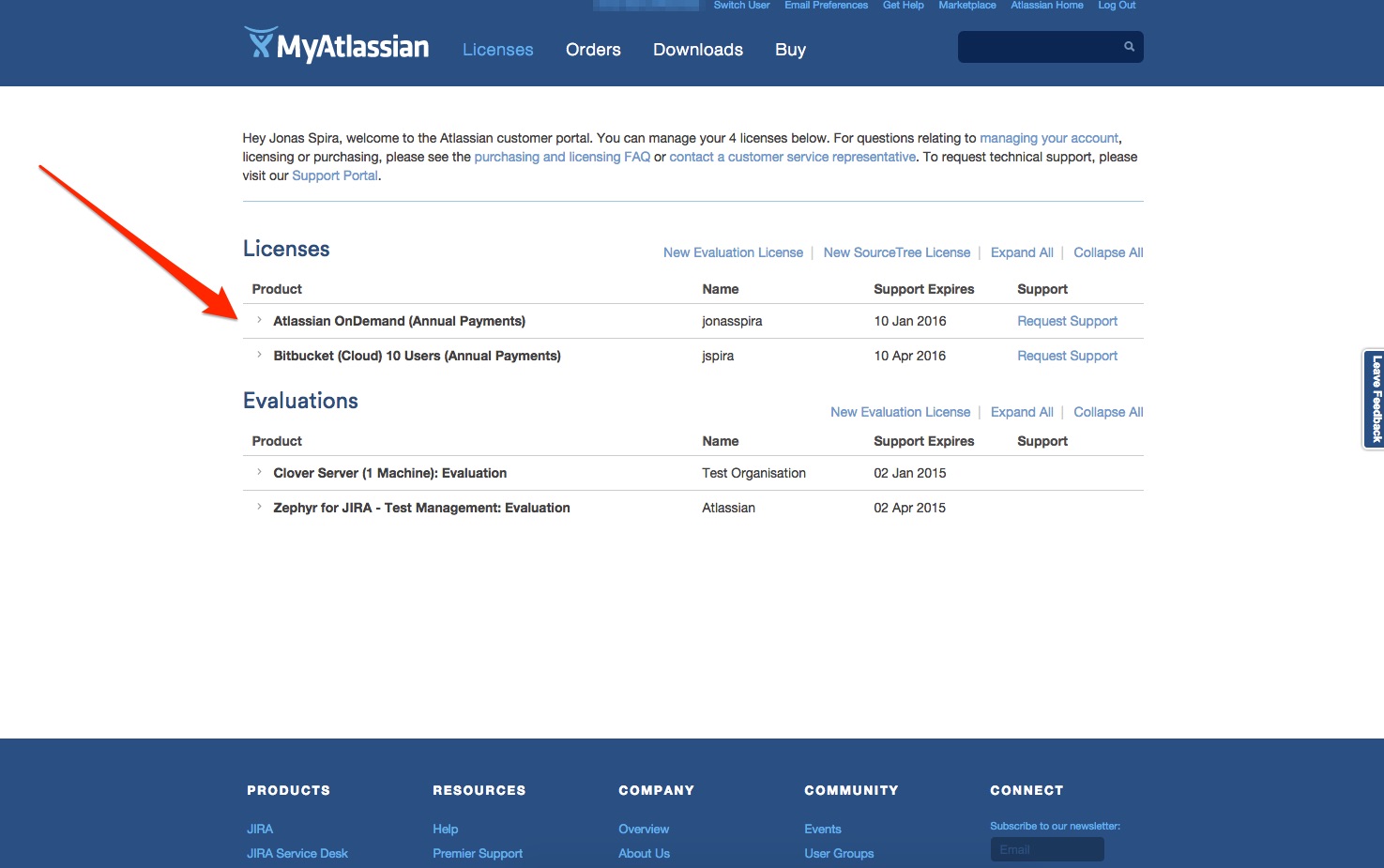The website interface features a predominantly white background with a blue header and footer. Centered at the top, the blue header contains the company logo, "My Atlatesian," with the logo in blue and the text in white. Below this, the header includes navigation options in blue and white font: "Licenses" (highlighted in blue), "Orders," "Downloads," and "Buy," along with a search bar on the right.

The main content welcomes the user, "Hey, Jonah Spira, welcome to the Atlantean customer portal. You can manage your four licenses below." It provides hyperlinks for common actions such as "managing your account," "purchasing and licensing FAQ," and "contact a customer service representative." For technical support, users are directed to visit the "support portal" link.

Detailed information about the licenses is displayed below. The license section lists the product "Atlatesian On Demand" with the payment type (annual payments), the associated name "JoSandra," and the support expiration date, "January 10, 2016." Next to the license details is a blue "Request Support" icon. There is also a section for evaluations under licenses.